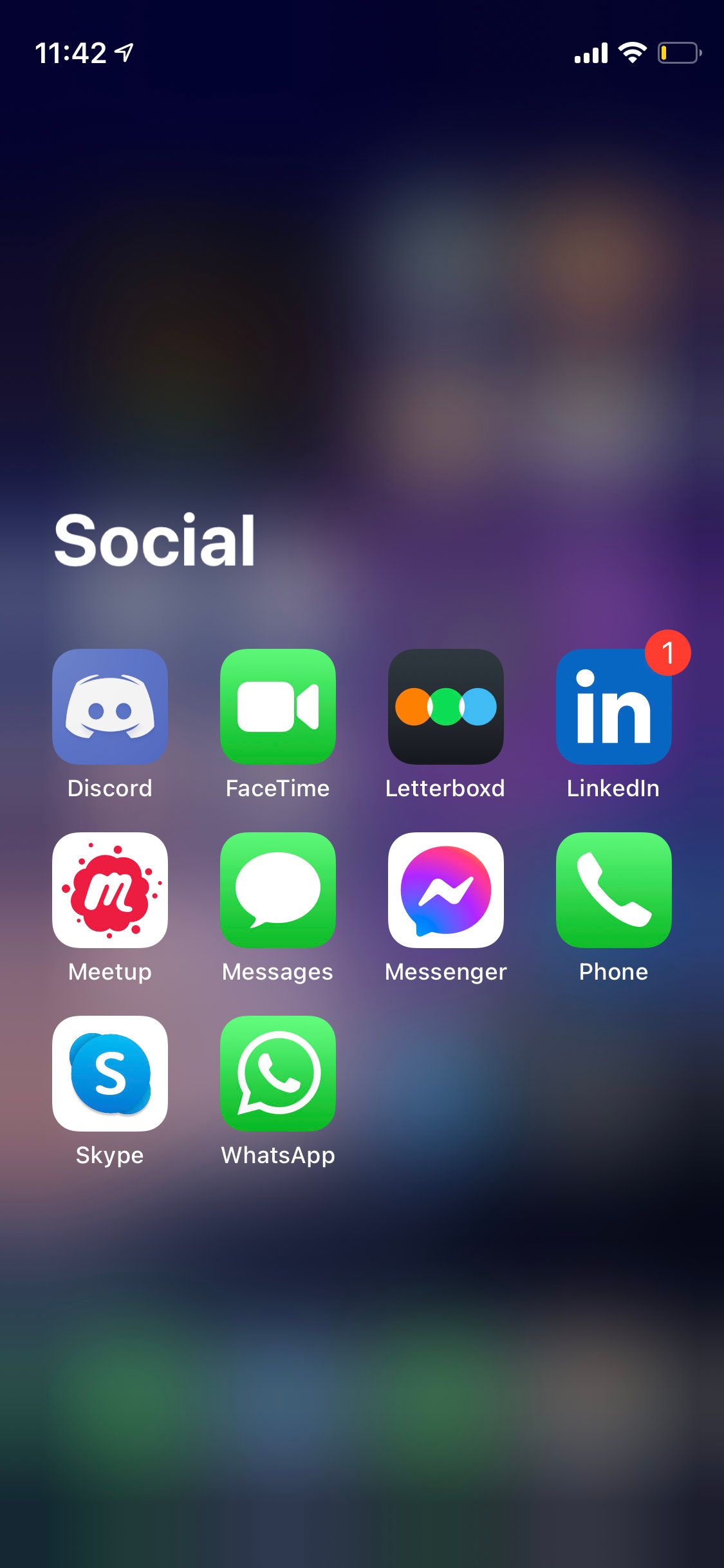The image captures a detailed screenshot of a smartphone's home screen, showcasing a well-organized array of app icons. At the top of the screen, the status bar displays the current time as 11:42. Adjacent to the time, the battery icon, colored yellow, signals a low charge level, alerting the user to recharge soon. Connectivity indicators display a strong signal with four bars and a connected Wi-Fi status.

The first row of app icons under a folder labeled "Social" includes Discord, FaceTime, Letterboxd, and LinkedIn, the latter distinguished by a small notification badge indicating the presence of one new message or update. 

In the second row, starting from the left, are the icons for Meetup, Messages, Messenger, and the Phone app. The third row features Skype and WhatsApp, each represented by their unique speech bubble icons.

The background of the screen appears slightly blurred, with indistinct colors blending together, emphasizing the clarity and prominence of the app icons. This organized and informative display provides a quick glimpse into the user's frequently accessed communication and social networking tools.